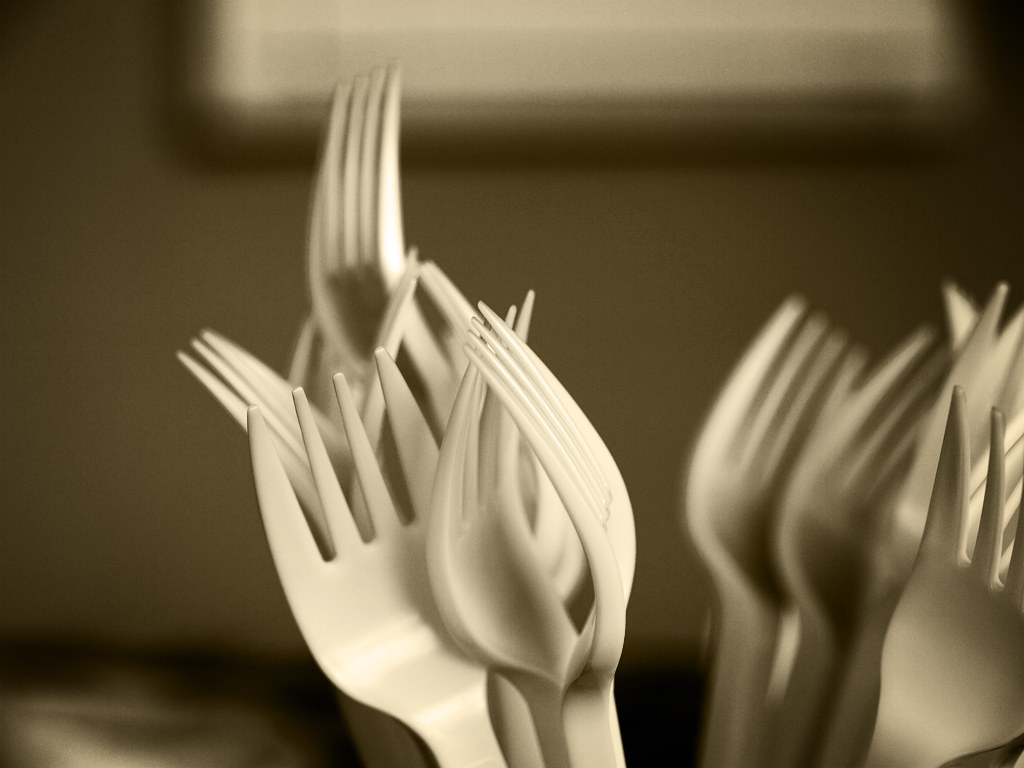The image is a slightly wider-than-tall, square photo featuring a detailed still life of upright white plastic forks in two distinct bundles. The background is heavily blurred, showing an off-white or tan wall with a hint of a wooden-trimmed window at the top. There are shadows cast to the right side, adding depth to the composition. The focus is primarily on the front cluster of about four forks, with one fork distinctly sticking up higher than the others. These forks are intricately tangled and leaning against each other. The bundles of forks vary, with one prominently in the center and another on the right-hand side. Both bundles display forks facing in different directions, intermingling within a likely unseen container. The overall effect presents a textured and dynamic arrangement, capturing the delicate interplay of light and shadow on the plastic surfaces.